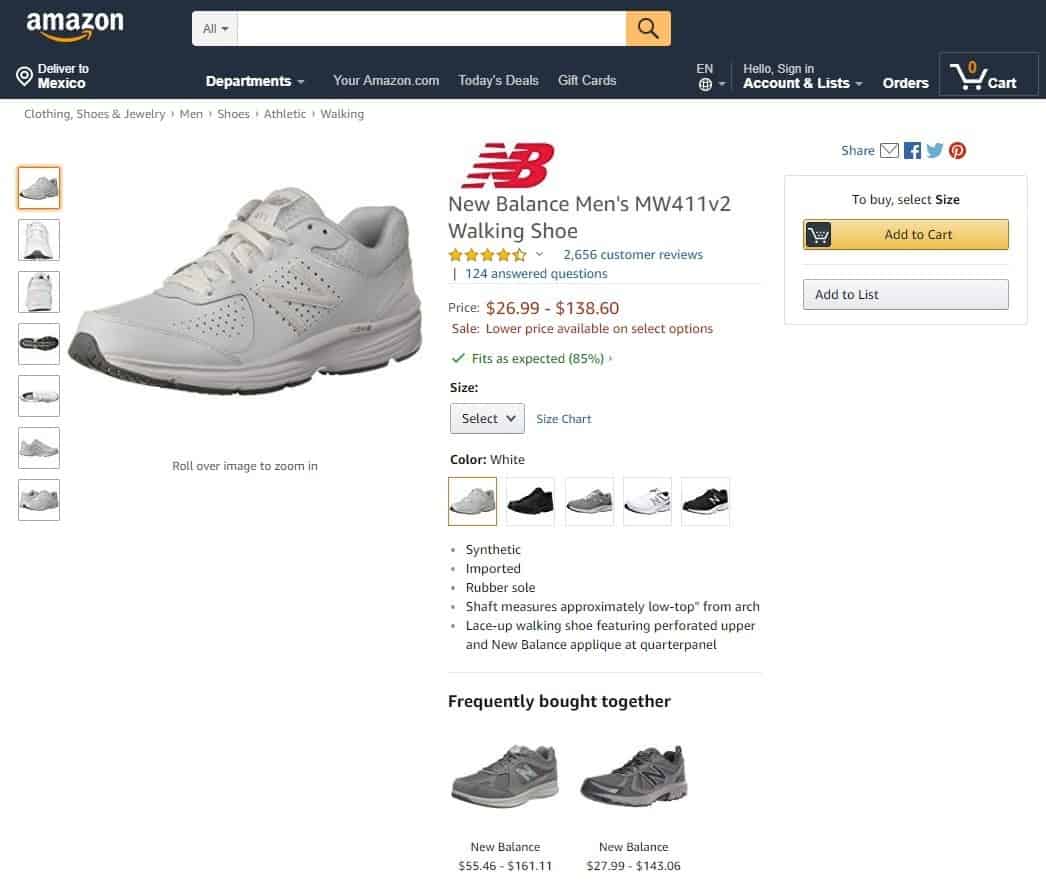The image is a screenshot captured from the Amazon website, showcasing the product page for the New Balance Men's MW411 V2 Walking Shoe. Prominently displayed in the center is a photograph of the shoe, with a series of smaller, clickable thumbnail images on the left side, allowing users to view the shoe from various angles. The customer rating is visible, with an average rating based on 2,656 reviews.

On the right, there are key interactive buttons, including "Add to Cart" and "Add to List," as well as sharing options via email, Facebook, Twitter, and Pinterest. The drop-down menus enable customers to select the shoe size, with an option to view a detailed size chart. Customers can also choose different color variants like white, black, and gray. 

The description indicates that the shoe is made of synthetic material, is imported, and features a rubber sole, with additional details such as shaft measurements provided. Below, there is a section listing items frequently bought together with the shoe. 

At the top of the webpage, the delivery location is set to Mexico. Navigation options for different departments, as well as links to sign in and view the shopping cart, are also available.